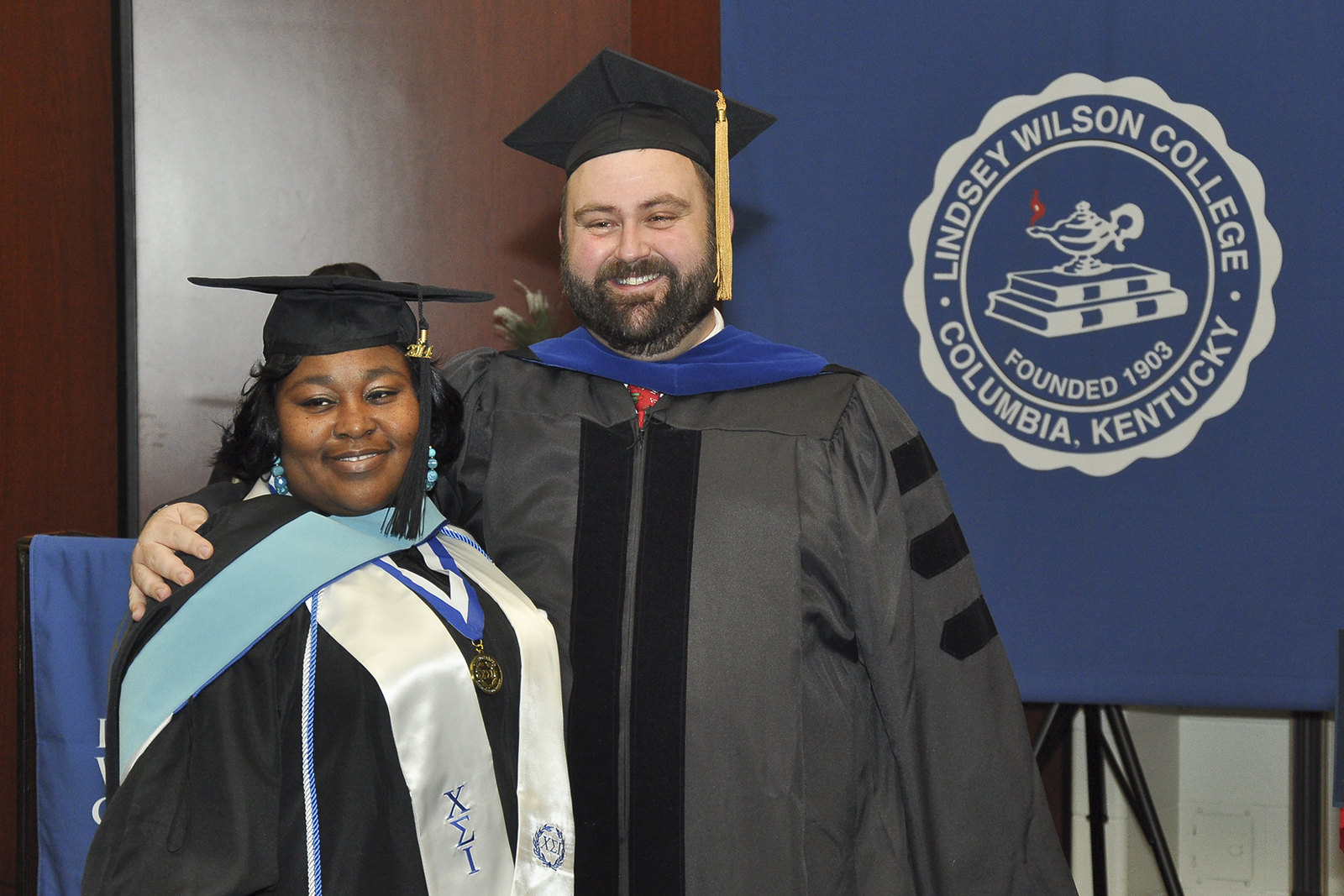This indoor photograph captures two individuals, a woman on the left and a man on the right, both dressed in black graduation robes adorned with various sashes and decorations. The woman, who has brown skin and black hair, is wearing an ornate gold medal over her chest along with white and light blue sashes. She is smiling but not looking directly at the camera. The man, with white skin and a very dark beard, stands beside her with his arm around her shoulder, also smiling. Behind them, there is a dark wood grain wall with a vertical black stripe on one side. To their right, a blue fabric sign on a black stand prominently displays the round white logo of Lindsay Wilson College. The logo includes an image of a stack of books with an oil lamp and the text "Lindsay Wilson College, Columbia, Kentucky, founded 1903" in white.